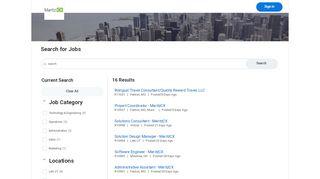This screenshot captures a job search website interface. In the top right corner, there's a blue button with white text. Below it, a full-width black and white banner showcases a cityscape of numerous high-rise buildings facing a bay. Below the banner, black text reads "Search for Jobs." 

On the left side of the webpage, there is a filter menu with sections titled "Current Search," "Job Category," and "Location." Users can check various tick boxes under "Job Category" to refine their search results. In the main content area, a user-entered search term has yielded 16 job listings. Each listing is displayed in blue font, with detailed job descriptions in black subtext.

In the top left corner, the search engine's logo is visible, starting with the letter 'M'.